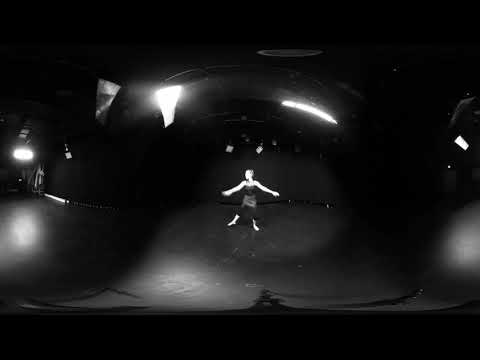The image is a horizontally oriented, rectangular photograph featuring a dark background with subtle variations in black and gray shades. At the very bottom, the image is almost entirely black, transitioning to darker gray areas as you move up. In the center stands a lone woman on what appears to be a hard-floored stage. She is dressed in a gray dress with black leggings and a black tank top. Her exact age and hair color are indeterminate, but her Caucasian features are discernible. She stands with her feet spread apart and her arms outstretched, giving the impression of a ballet or dance performance. Above her, the stage lights create abstract splotches, one resembling a funnel and another like a dash, bending and warping in a visually distorted manner. The scene is lit with black, white, and different shades of gray, contributing to an eerie, surreal atmosphere. Despite the distortion, the setting clearly depicts an indoor stage during a live performance, emphasizing the solitary dancer's poised stance amidst the warped brilliance of the stage lights.